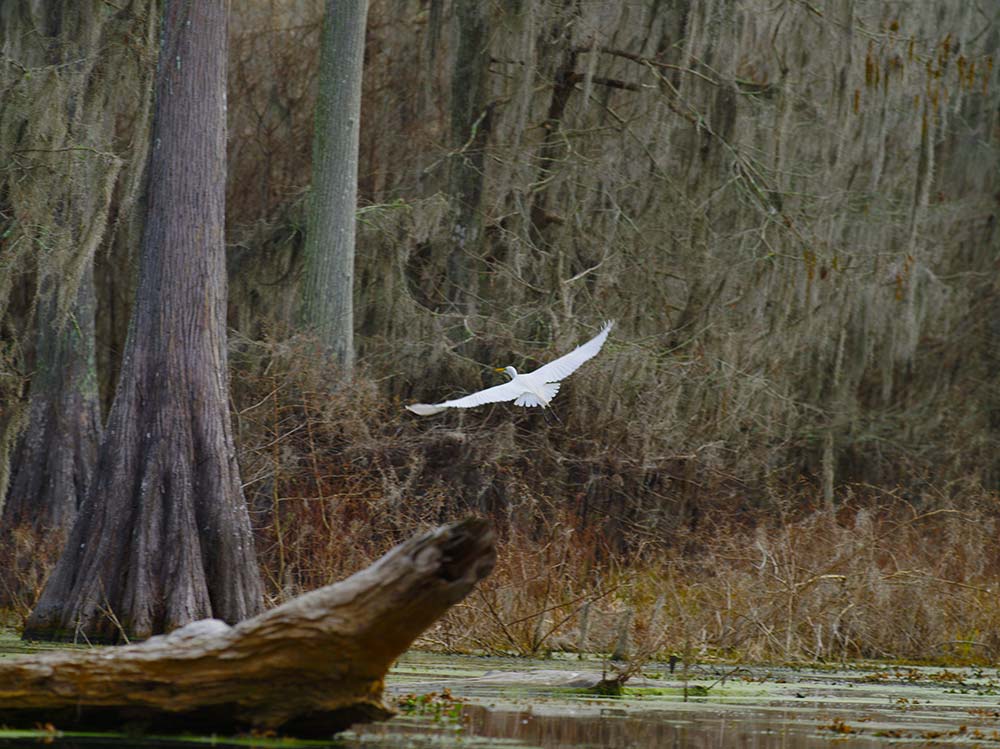The image depicts a vibrant white bird with fully stretched wings, flying leftwards over a swampy area. The bird, characterized by its thin neck, long wings, yellow beak, and gray legs, contrasts vividly against the murky brown and green water below, which is interspersed with lily pads, green slimy moss, and floating dead leaves. A large fallen tree trunk, covered in green moss, occupies the lower left of the photo, while other similar tree trunks and stumps, partially submerged, are scattered throughout the scene. Prominently on the left, a large tree with a wide base and slim trunk rises from the swamp, its dark gray bark stark against the backdrop. In the distance, more trees draped with hanging gray Spanish moss line the area, contributing to the dense and natural atmosphere. The grasses and plants surrounding the water are a mix of brown and green, indicating a rich and diverse ecosystem. The moving water suggests this is part of a river rather than a stagnant pond. Overall, the image captures a dynamic and lush swamp teeming with life and natural elements.